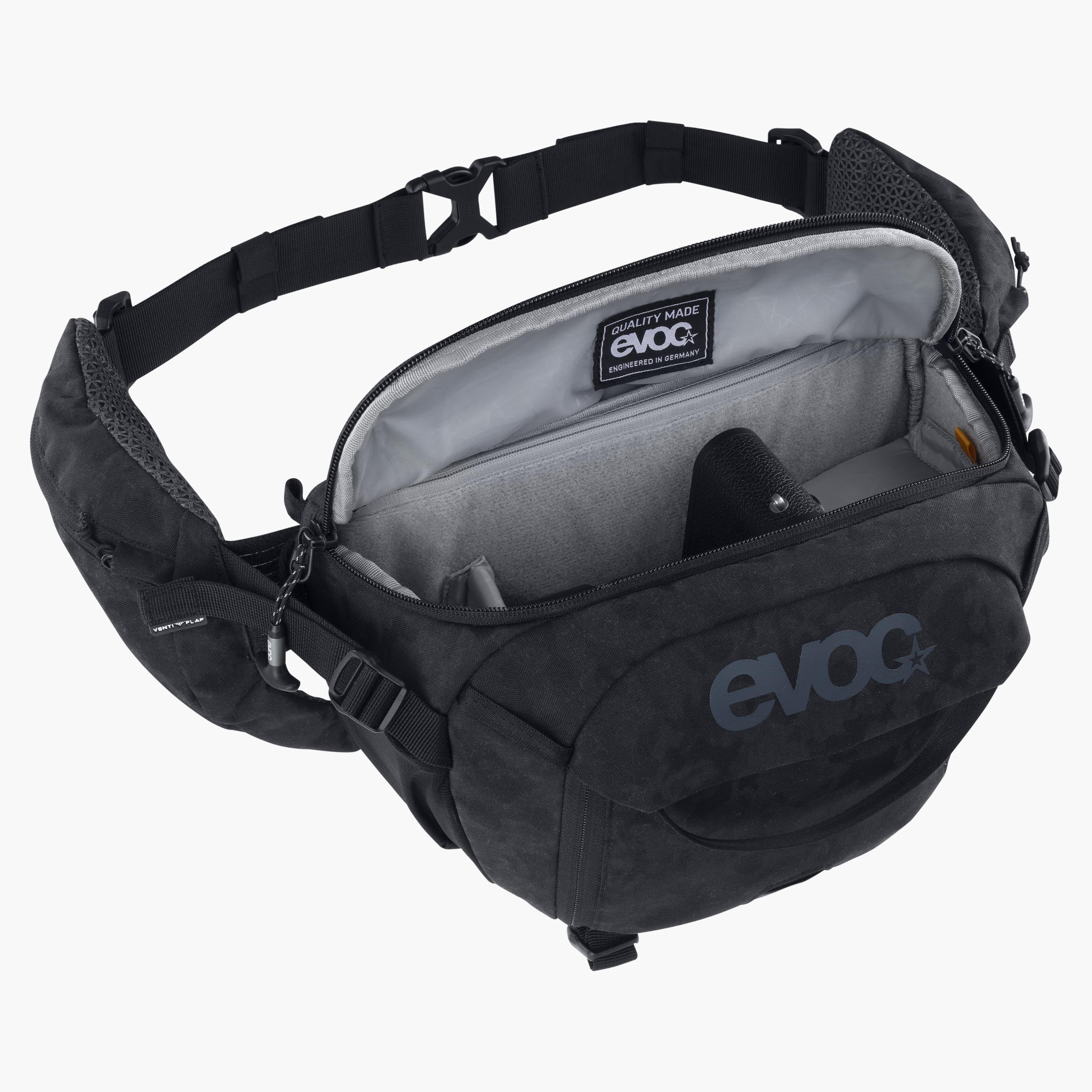This image depicts a compact, dark-colored nylon bag, resembling a small duffel bag. The exterior is primarily dark gray, almost black, and features a prominent logo that reads "EVOC" on the front. The bag is equipped with a shoulder strap, providing convenience for carrying. The interior contrasts with a light gray lining, offering a stylish interplay of shades. Despite its diminutive size, this bag appears functional and versatile, suitable for storing essential items.